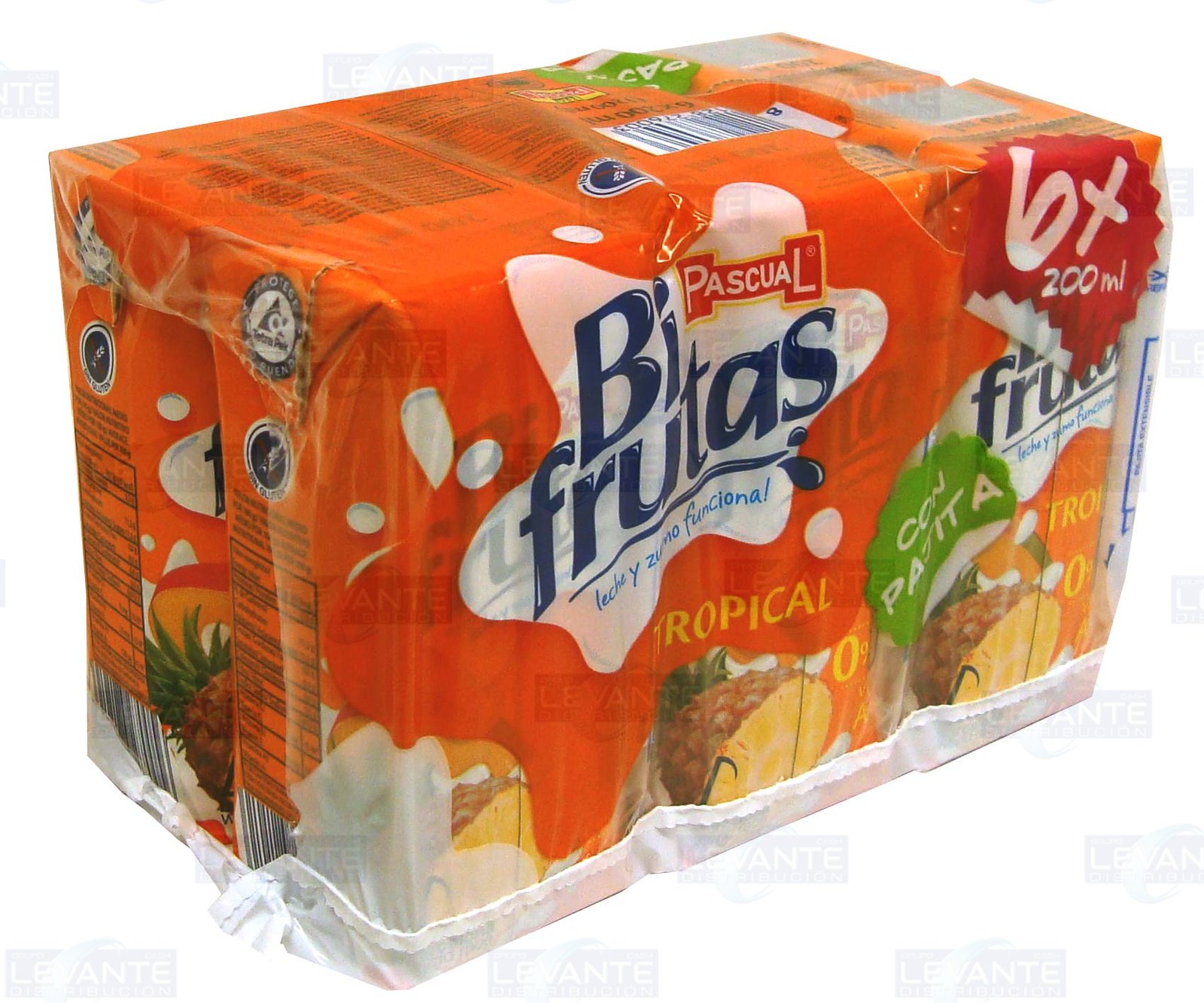This image features a professionally photographed stock photo of a six-pack of tropical fruit punch juice cartons, designed against an all-white background, suggesting an advertisement style. Each carton is encased in bright orange plastic packaging adorned with Spanish text, including phrases like "buy frutas" and "tropical." The prominent images of pineapples on the packaging indicate the juice's pineapple flavor. The cartons, which are tall and rectangular in shape rather than traditional juice cans, also display some decorative elements and possibly nutritional information, although the latter is not clearly visible.